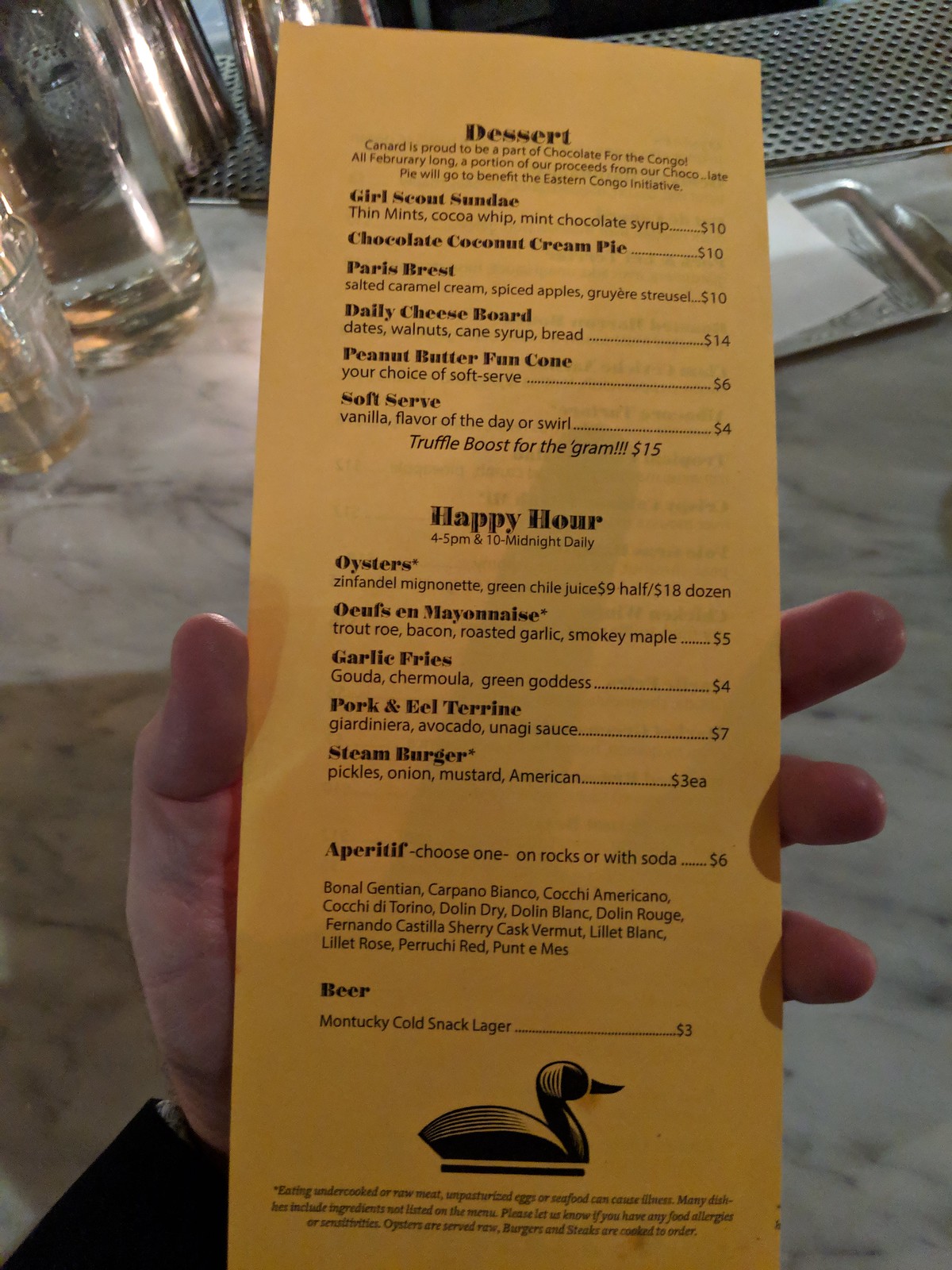This is a photograph of a brightly colored menu, held vertically in someone's left hand, prominently displayed in front of the camera. The background showcases elegant glasses placed on what appears to be a sleek, polished marble countertop, adding a touch of sophistication to the scene.

The menu itself is eye-catching with its yellow backdrop and contrasting black typeface. It is neatly organized into various categories, including a dessert section offering a delightful array of sweet treats such as Girl Scout Cookie, Chocolate Coconut Cream Pie, Paris Breast, a variety of cheese boards including a Daily Cheese Board, Peanut Butter Fun Cone, and Soft Serve Ice Cream. The prices for these desserts range from $4 for the Soft Serve Ice Cream to $14 for other delectable options.

Additionally, there is a Happy Hour menu featuring an enticing selection of items such as Oysters, a dish coupled with Mayonnaise, Garlic Fries, Pork and Eel Terrine, and a Steam Burger. These items are priced attractively between $3 and $5, perfect for a casual yet refined dining experience.

The menu also includes a selection of aperitifs and beers, with the aperitif priced at $6, providing a perfect prelude to a meal or a standalone indulgence.

Notably, at the bottom of the menu, there is a charming image of a duck, adding a unique and playful element to the overall menu design. Although some prices are slightly challenging to discern due to the small size of the image, the clear categorization and intriguing offerings make this menu inviting and appetizing.